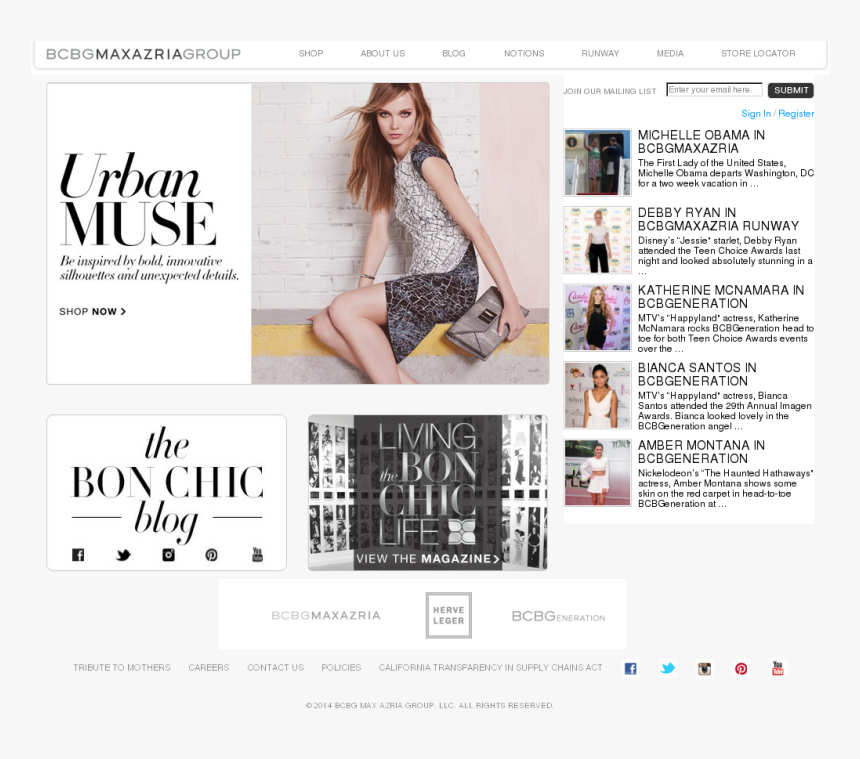The image is a screenshot of a website with a white background. At the very top is a white navigational menu. The upper left-hand corner features the company's name, "BCBG," in gray font, followed by "MAXAZRIA" in black font, and "GROUP" in gray font.

Centrally located near the top of the page is a photograph of a model. She is a very thin white woman with long red hair that nearly reaches her elbows. She is wearing a dress with a silver top half and a darker silver-gray bottom half that falls a little above her knees. The model is sitting down and looking directly at the camera.

To the left of the model, there is a dark gray headline reading "Urban Muse." Below the headline, a subtext in a smaller font states, "Be inspired by bold, innovative silhouettes and unexpected details."

On the right side of the website, there are several news items, represented by five photos stacked vertically. The top photo features Michelle Obama.